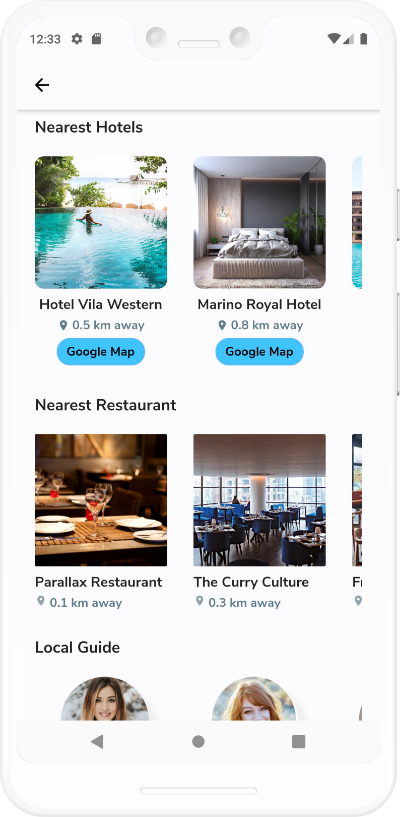The image depicts a mobile app designed to showcase nearby hotels and attractions with a user-friendly interface. The app's layout resembles an iPhone with a notch at the top but hints at a possibility of being on an Android device. The primary screen prominently features professional and visually appealing photographs of two hotels: the Hotel Villa Western and the Merino Royal Hotel. Notably, both hotels are conveniently situated within a mile from the user’s location.

Beneath the hotel listings, a Google Maps button is visible, enabling users to easily access directions to these accommodations. The app also includes a section dedicated to nearby restaurants, mentioning the Parallax Restaurant and The Curry Culture, both within a half-mile radius.

The interface highlights local guides as well, with images of two young women who appear to be part of this section, although their exact roles remain unclear. The overall design benefits from a clean, white background, ensuring that text and images are easy to read and navigate. This app serves as a handy tool for users to explore and find local amenities and attractions efficiently.